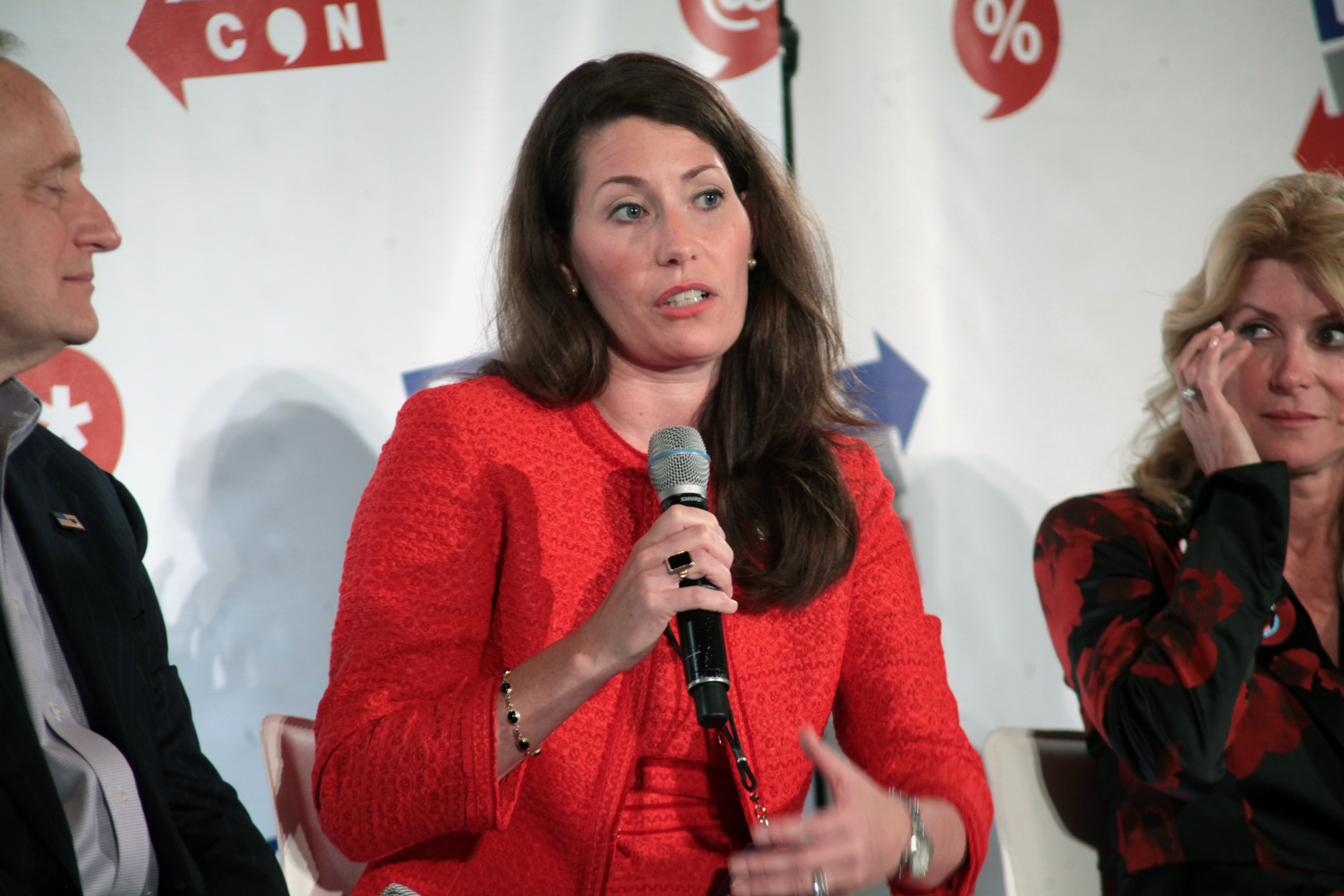In this image, three individuals are positioned in front of a white background adorned with a partially visible poster. The poster, which appears to be for a public event or conference, features several colorful arrows and various symbols, including the letters "C-O-N" inside a red arrow that points to the left, as well as a percent sign, an asterisk, and an at sign.

At the center of the image, a woman in a red dress or jacket (which matches her reddish lipstick) is holding a gray-headed, black microphone while seated, likely answering questions. Her chest-length black hair frames her face, and she is adorned with jewelry, including earrings, a bracelet, a silver wristwatch, and a wedding ring. She is looking to her left, revealing her teeth as she speaks.

To her right (the viewer's left) is a man attentively gazing at her. He is dressed in a black suit jacket, which is accented with an American flag pin, and he dons a white button-down shirt underneath. 

On the woman's left (the viewer's right) is another woman wearing a black and red dress with a floral print. This woman has shoulder-length blonde hair and appears to be wiping her eye. All three individuals seem to be deeply engaged in the moment, suggested by their focused expressions and postures.